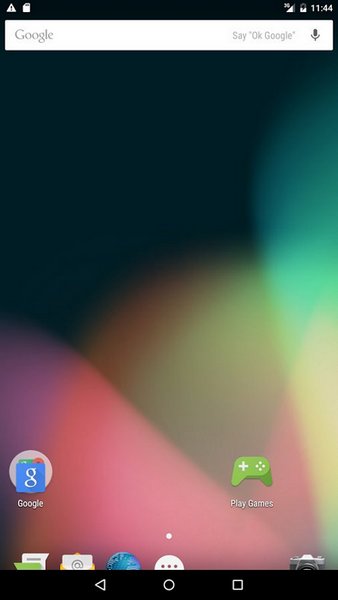This image appears to be a screenshot of an Android home screen. At the very top, a series of icons are displayed, though their meanings are not immediately clear to the observer. Among these icons is one featuring a triangle with an exclamation mark inside it, alongside another that resembles a book with a dog-eared page. The screen indicates the time as 11:44. Additional icons suggest the user might have headphones connected, as well as another unidentified icon.

Prominently situated at the top of the screen is the Google Search bar, complete with the Google logo on the left and a microphone icon on the right, inviting the user to "Say OK Google" for voice commands. 

The lower portion of the screen showcases a variety of app icons. Specifically, from left to right there are icons for Google, Play Games, Camera, and a browser represented by a globe icon. Three other partially visible icons remain towards the bottom edge: one depicting a circle with three dots, another representing an email app featuring a yellow envelope with an '@' symbol, and the last one displaying two overlapping pieces of paper, with one piece colored green.

Finally, along the bottom edge of the screen, the navigation bar features the standard Android controls: a triangle for "Back," a circle for "Home," and a square for "Recent Apps."